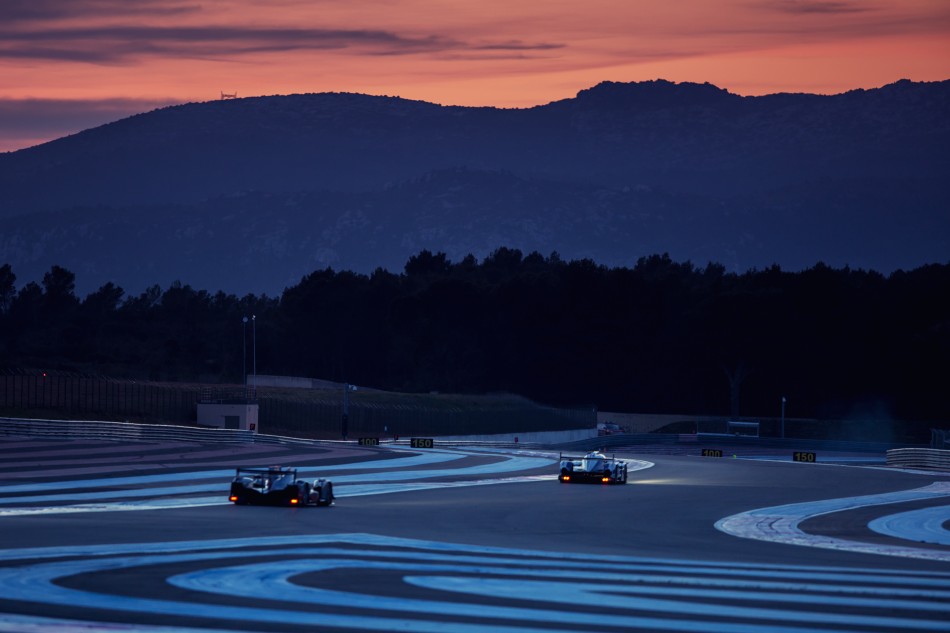The image depicts a dramatic F1 race taking place at dusk on a winding racetrack. In the foreground, two sleek, all-black race cars, with their powerful headlights piercing the growing darkness, are captured speeding from the bottom left to the middle right of the frame. Their rear lights glow vividly as they navigate the intricate course, defined by white flowing lines. The racetrack itself is highlighted in the bottom third of the photo, providing a clear path amidst the action.

In the middle distance, a dense green forest of tall trees creates a natural barrier, adding to the scene's depth and texture. Beyond the forest lies a series of imposing rocky hills, their outlines softened by a layer of mist drifting to the right. These hills, covered partially with trees, appear dark and brooding under the evening sky.

The background showcases a recently set sun, casting a vibrant palette of oranges, pinks, and reds across the sky. Light streaks of thin, black clouds stretch predominantly from the left, adding to the moody atmosphere. Further enhancing the scene is a conspicuous small shed, nestled within the middle ground, and numerous unlit lights. Signs with numbers and directional arrows are also visible, guiding the racers through the turns of the track. The entire scene captures the essence of an exhilarating evening race amidst a picturesque, yet slightly ominous, natural setting.